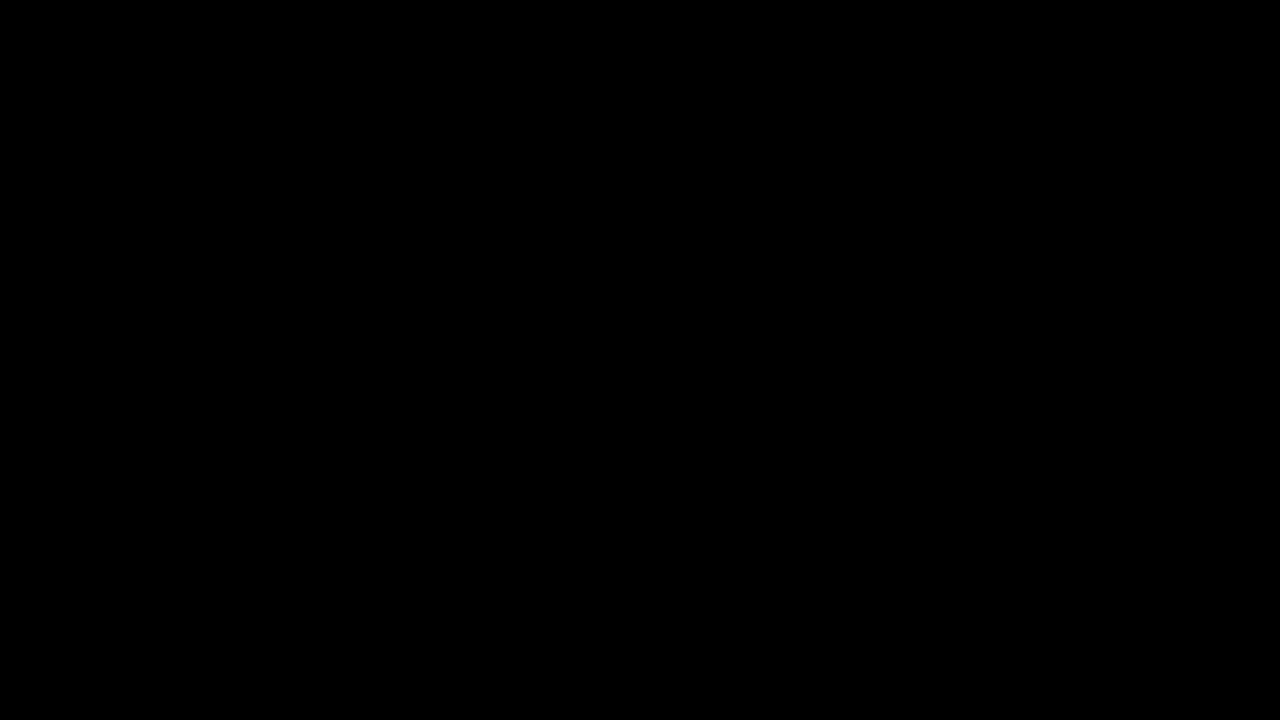The image in question is a completely black rectangle with no discernible elements, features, or variations. It contains no logos, characters, words, or numbers—just a uniform monochrome black color extending across the entire image. Resembling a blank slate or a dark room with no light, it gives an impression of absolute darkness. This could be intentional or possibly an error, but regardless, the image is devoid of any details or overlays.